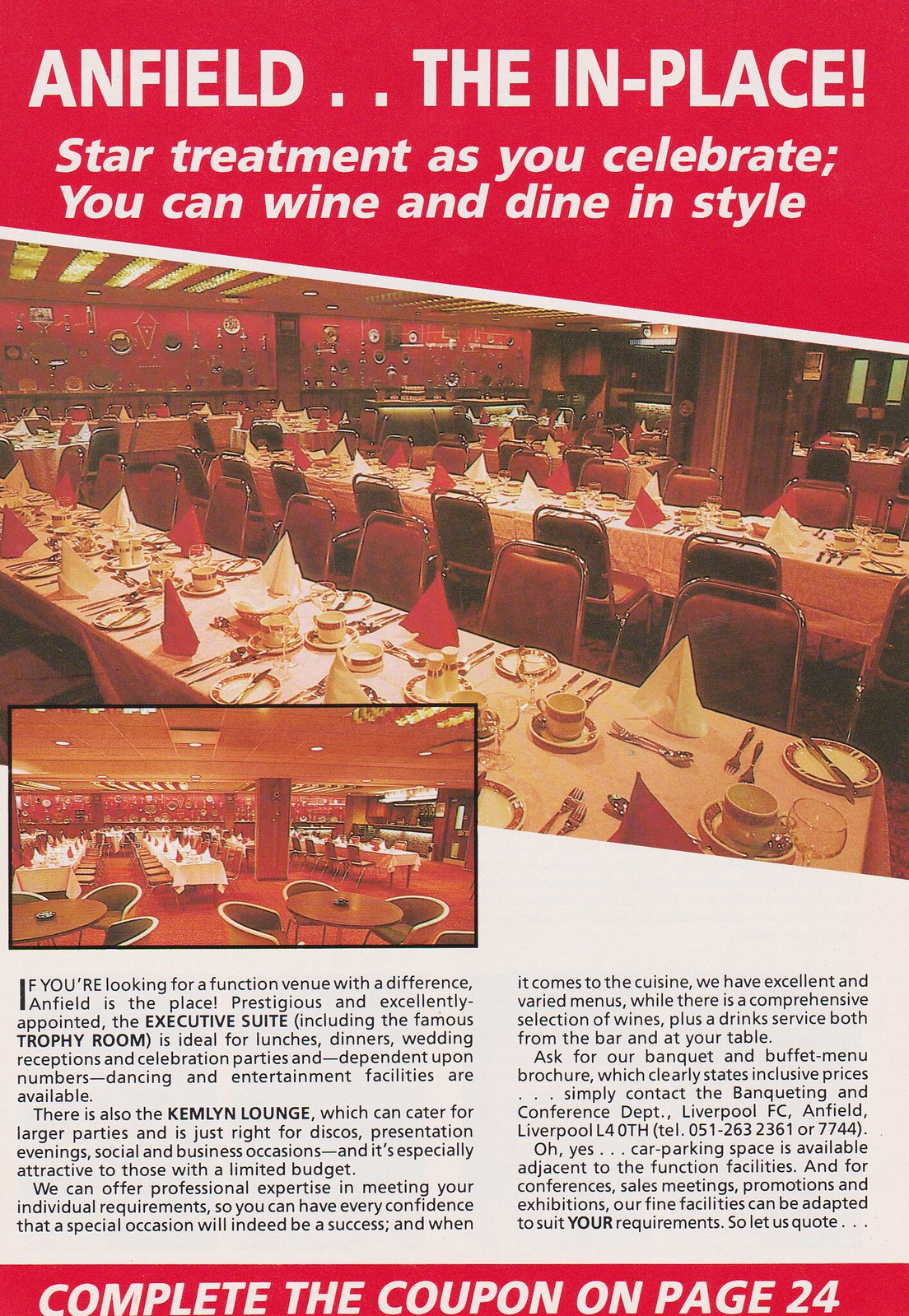This vertically aligned rectangular image resembles a magazine page. The top section has a striking red background with large white all-caps text that reads, "ANFIELD... THE IN PLACE!" Below that, in smaller white lowercase letters, it states, "Star treatment as you celebrate. You can wine and dine in style." A diagonal white line separates this section from the middle portion of the page, which showcases an image of a lavish dining setup. Long rectangular dining tables are adorned with alternating red and white cloth napkins standing upright. The tables are set with coffee cups on saucers, silverware, and dinner plates. The red-backed chairs with metal outlines enhance the elegance of the arrangement. A smaller inset image on the left side displays round tables with rounded-back chairs, indicative of a different section within the same room, as the long rectangular tables are visible in the background. The bottom part of the page includes two columns of text on the left and right, with several paragraphs that likely describe the venue and services. Finally, against a red background at the very bottom, the text emphatically instructs, "COMPLETE THE COUPON ON PAGE 24" in all-caps white letters.